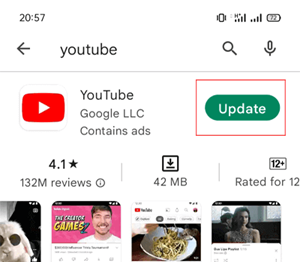The image is a screenshot of the YouTube application page from a mobile device's app store, displayed against a solid white background. At the top left corner, the current time is shown as 20:57. On the top right, there are icons indicating the phone's signal reception and battery status, which is at 72% charge.

Below this, there is a horizontal row containing a back arrow button on the far left, followed by the text "YouTube" in black, a magnifying glass icon representing the search function, and a speaker icon on the far right, likely for audio settings. A thin gray horizontal line separates these elements from the rest of the screen.

Underneath this line, the YouTube logo is displayed on the left side in a light gray box. The logo consists of a red rectangle with a white play button symbol in the middle. To the right of the logo, "YouTube" is written in gray text, followed by "Google LLC."

Continuing down the screen, there is a line of text that reads "Contains ads" in gray. To the right of this text is a red rectangle border containing a green "Update" button. Below this section, there is a black star rating of 4.1, followed by the text "132M reviews." To the far right, the download size is listed as "42MB."

This detailed caption provides a comprehensive description of the app store screenshot for the YouTube application.